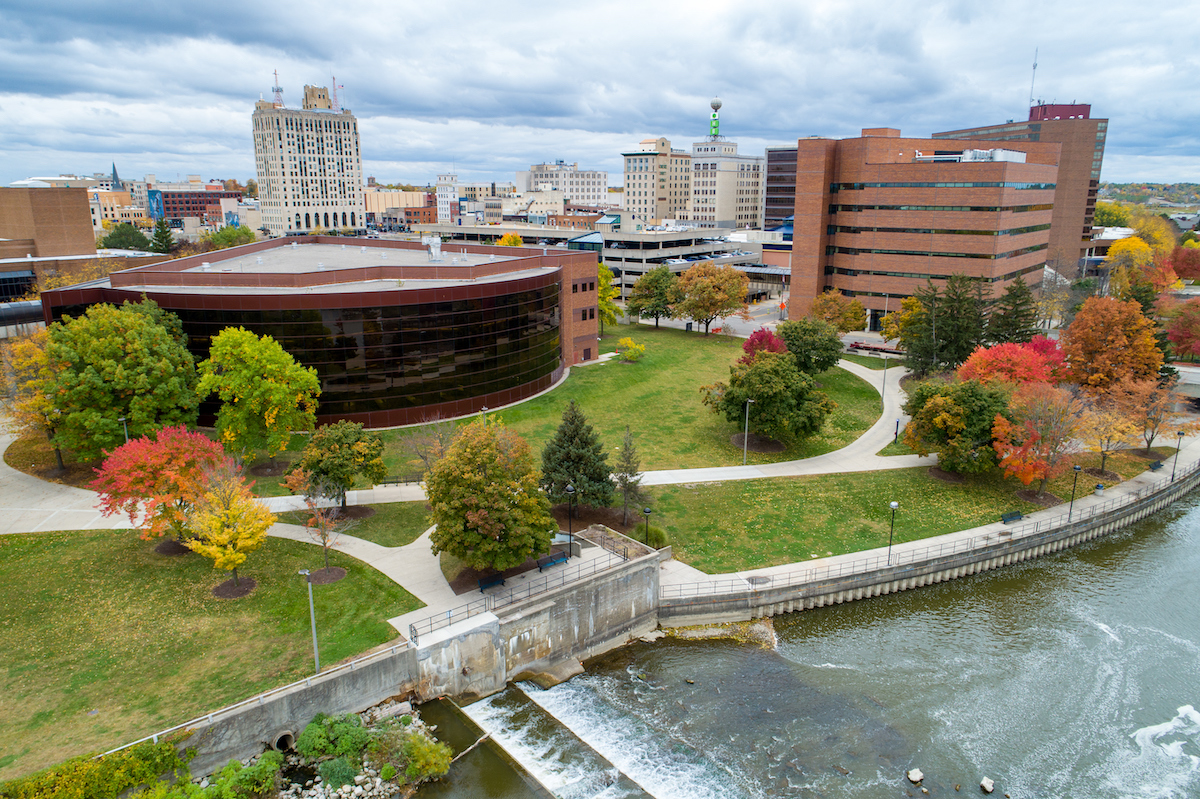The image captures a vivid view of a bustling downtown area from a high vantage point, possibly a 10-story building's balcony, looking across a murky, flowing river segmented by low barrier dams. The water cascades over these barriers, producing white water rapids. A concrete wall with sidewalks runs parallel to the river, stretching from the lower left to about midway on the right of the image, leading into a well-maintained park area. This park features greenish-brown grassy lawns, park benches, and thick sidewalks, interspersed among a variety of tall trees. The deciduous trees display a colorful array of green, orange, yellow, and red leaves, signaling autumn, with only a single evergreen standing out.

The closest structure is a distinct brown brick building with a rounded wall of dark glass windows facing the river. Nearby, to the upper right, there is another brick building approximately eight or nine stories high. This urban backdrop includes additional notable buildings such as a concrete parking garage and several mid-rise skyscrapers, all contributing to the dense cityscape. The skies above are gray and cloudy, lending a subdued but bright atmosphere to the scene.